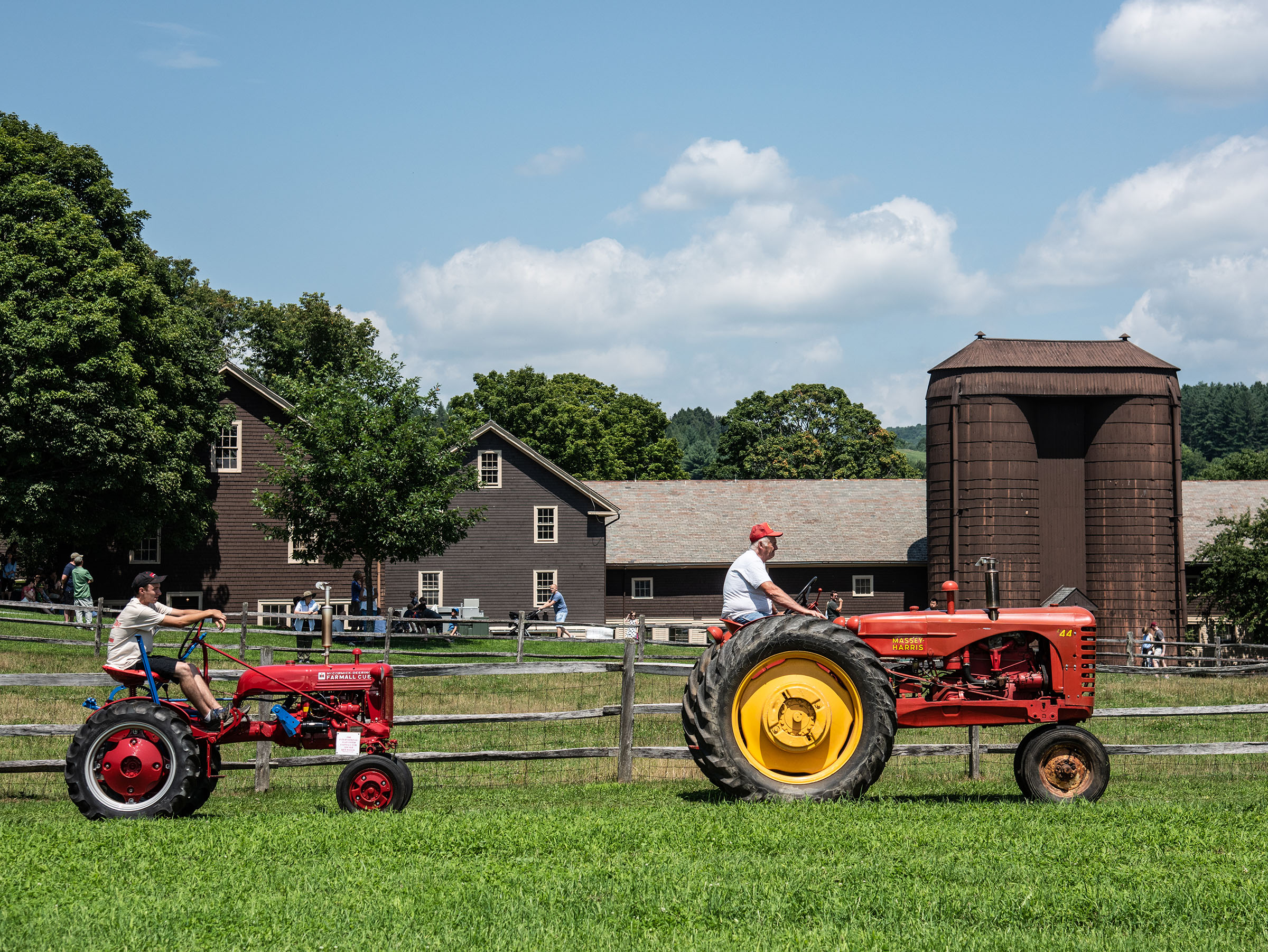This image captures a vibrant, bustling farm under a bright, sunny sky adorned with fluffy white clouds. In the foreground, lush green grass stretches towards a wooden fence with three planks and sturdy posts, which separates two red tractors. A man wearing a red cap sits on the larger tractor, distinguished by its bright yellow back wheels and smaller black front wheels. Nearby, a boy clad in a white shirt and black shorts rides a smaller red tractor with two big back wheels and smaller front wheels. Behind the tractors, the scene extends to a lively backdrop where groups of people are engaged in various activities. Some are lounging under a tree, others play baseball in a field, while a few roam near the silos and stables. The farm's central structure is a sprawling grey farmhouse with white-framed windows, featuring both one-story and multi-story sections. Surrounding the farmhouse is a tree line that merges seamlessly with the blue sky, completing the picturesque rural setting. The tractors bear visible text in contrasting colors—white on the smaller one and yellow on the larger one—adding a subtle touch of detail to this high-quality, panoramic snapshot of farm life.